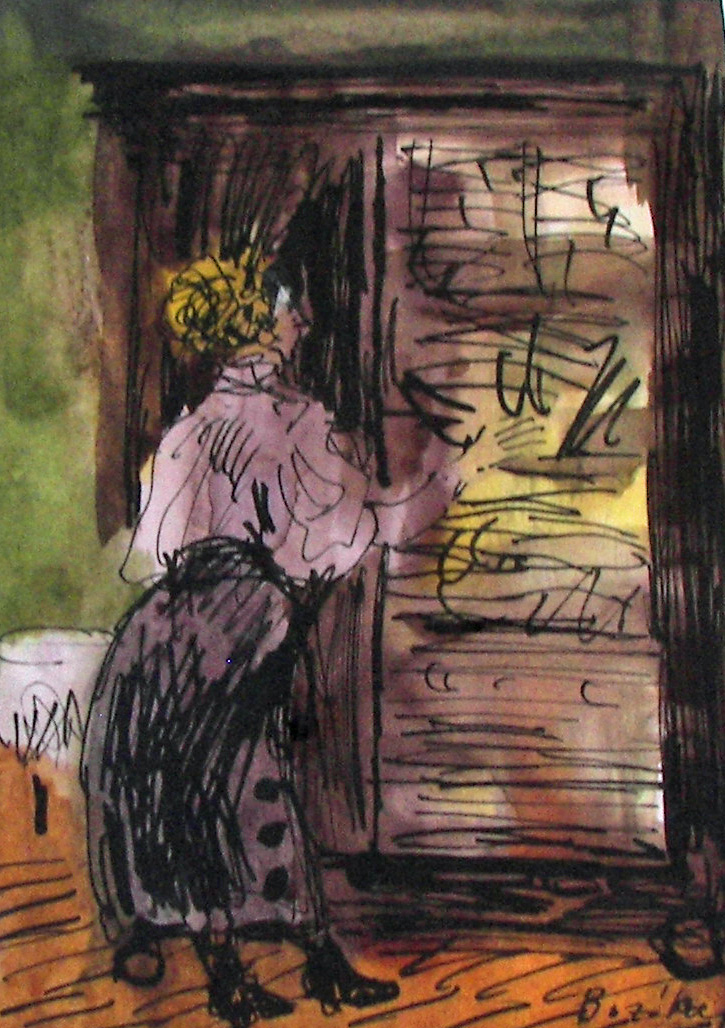This vertical rectangular painting features a woman with her back to the viewer, poised before a large cabinet. She has blonde hair with black streaks, styled in curls and pulled up. Her attire consists of a purple blouse and a matching skirt adorned with black squiggly lines, adding a distinctive texture. The woman is depicted with one arm extended toward the cabinet, suggesting an interaction with it.

The cabinet itself is primarily purple with segments of yellow and white, detailed with black squiggly lines that create a sense of movement and depth. To the left of the cabinet, there's a small round white table covered with a white tablecloth. The floor beneath is brown with black scribbles, and the wall in the background is green, also accented with black lines, giving the composition a cohesive, scribble-centric artistic style.

This painting, likely a watercolor due to its fluidity and texture, is signed in the bottom right corner, possibly with the name "Buzoki" or "Bozekes." The overall style appears to blend traditional motifs with abstract, scribbled detailing, creating an intricate and engaging scene.